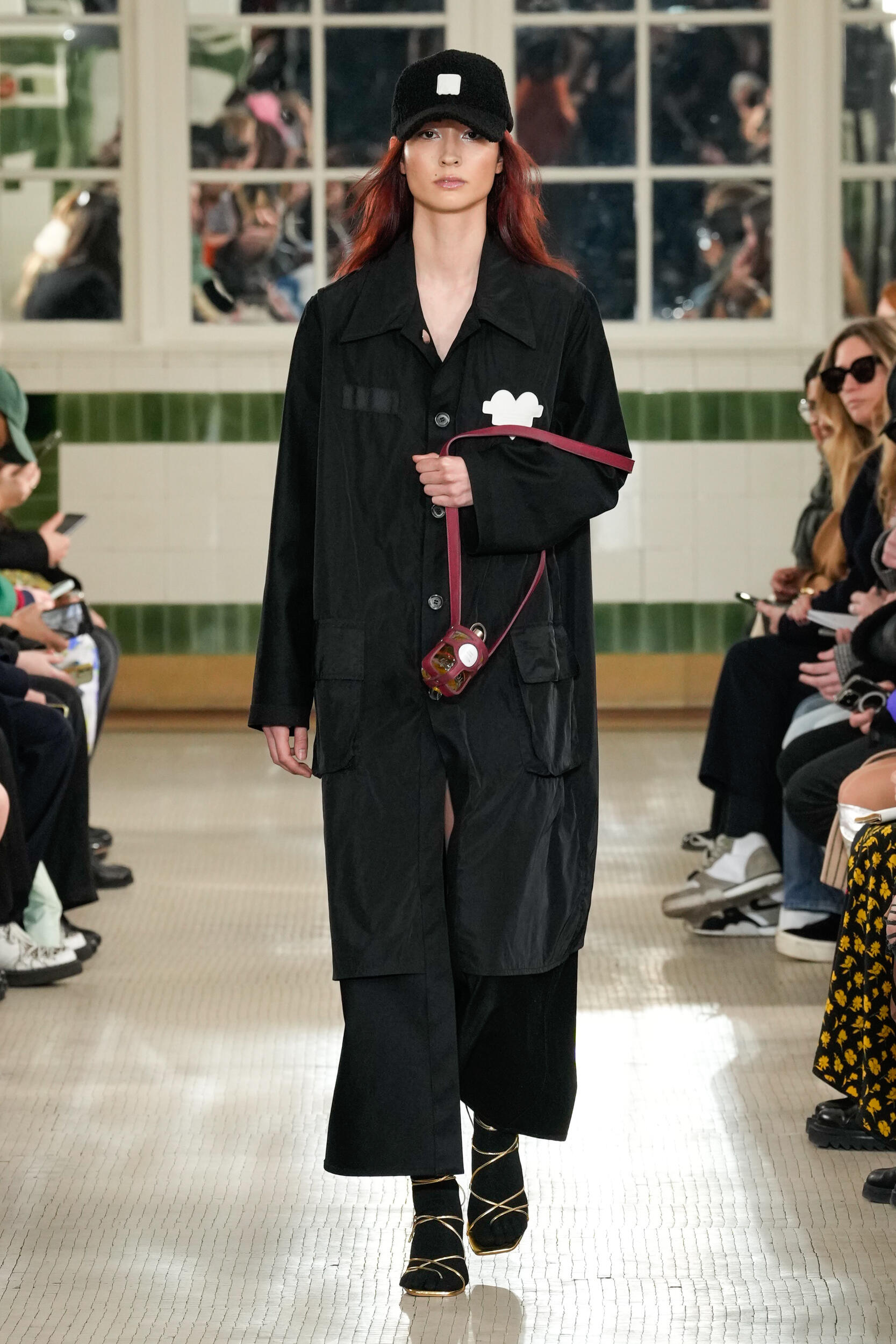The photograph captures a female model confidently striding down a catwalk during a runway fashion show, surrounded by an audience lining the aisle. The model, who appears to be of white, possibly Hispanic or Asian descent, is the focal point of the image. She has distinct reddish or auburn hair that peeks out from under a black baseball cap featuring a white square emblem. Her expression is deadpan, contributing to the high-fashion ambiance of the scene.

She is adorned in an almost entirely black ensemble, consisting of a loose-fitting, trench coat-style top with a noticeable white heart logo crossed by a thick line at chest level. Complementing the top are long black pants that end at her ankles, black socks, and striking gold strappy sandals that intriguingly weave between her toes even with the socks on. Adding a pop of color to her monochromatic outfit, she holds a unique, small red strap bag that dangles by her left hip, resembling a carabiner or a compact case. The background blurs out, emphasizing the model's poised figure and the intricate details of her outfit, highlighting the event's chic and meticulously curated atmosphere.